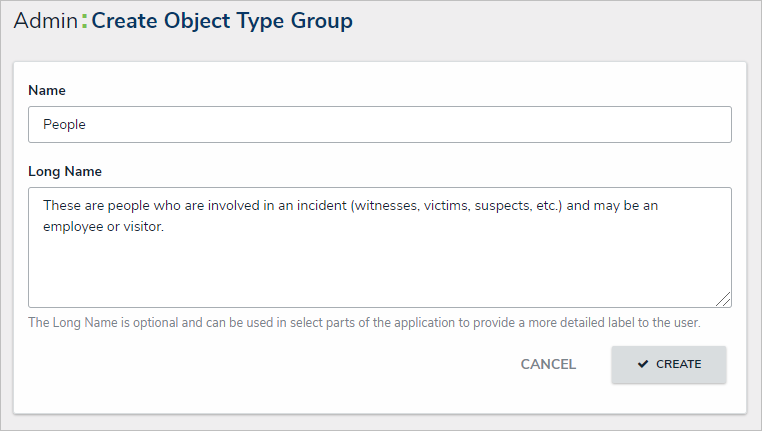**Caption:**

This image captures a computer screen displaying an admin interface for creating an object type group. The screen's backdrop is a muted gray, while the main content is housed within a crisp white rectangle.

At the top of the screen, the title "admin: create object type group" is displayed in different colors: "admin:" in black with a green colon, followed by "create object type group" in navy blue.

Within the white rectangle, the interface prompts the user to input details for the new object type group. First is a field labeled "Name" with an accompanying text box, currently filled with the word "people." Directly below, another field labeled "Long Name" contains the phrase: "These are people who are involved in an incident (witnesses, victims, suspects, etc.) and maybe an employee or visitor."

The lower section of the screen includes a note indicating that the "Long Name" is optional and may be used throughout the application to provide a more detailed user label. At the bottom, there are two clickable options: a gray "Cancel" button and a blue "Create" button.